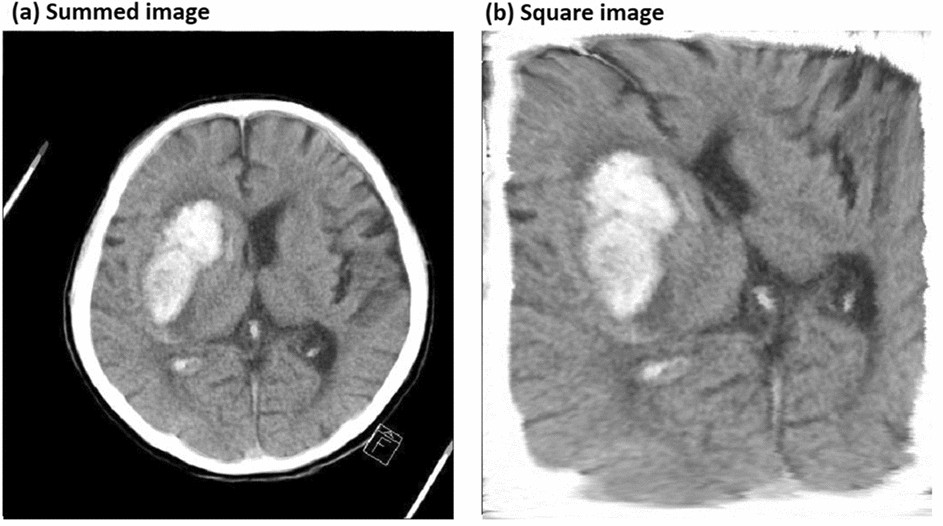The image consists of two side-by-side brain scan pictures, each with a white background and labeled in black font. The left picture, labeled "A summed image," features a circular scan that shows the brain's gray matter with notable squiggly lines and white patches. The right picture, labeled "B square image," is a zoomed-in, square version of the same brain scan. This zoomed-in view highlights the gray matter in more detail, with white areas and black, shiny spots that resemble small beads. Both images have blurred borders, with the right image presenting a closer look at the brain’s intricate structures.